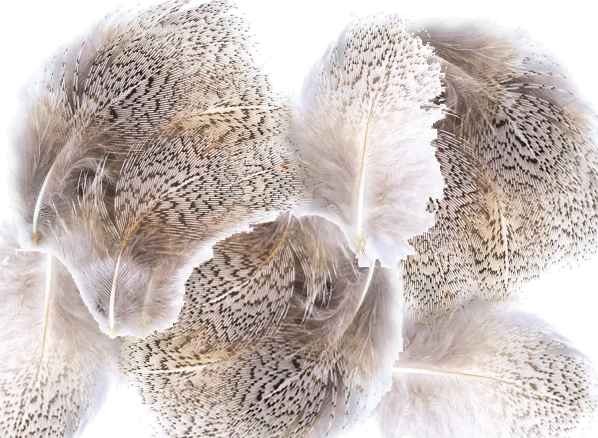This is a highly detailed, digital artwork depicting a randomized pattern of bird feathers. The feathers, primarily colored in various shades of brown, feature intricate black speckles that add texture and depth. They transition in color towards the tips, displaying lighter gray and black stripes. Each feather is outlined with a slightly pixelated white border, and some even have a white central vein. These feather elements vary in shape and size, reminiscent of both down feathers and larger, flight feathers, creating a sense of lightness and fluffiness. They are overlaid multiple times, rotated, and arranged in an abstract, almost dreamlike composition with varying degrees of opacity and a subtle white glow emanating from behind. The overall effect is an artistic and ambiguous visual, lacking any text or defining annotations, inviting viewers to interpret the scene as either a realistic close-up of bird feathers or as an abstract, three-dimensional illustration.